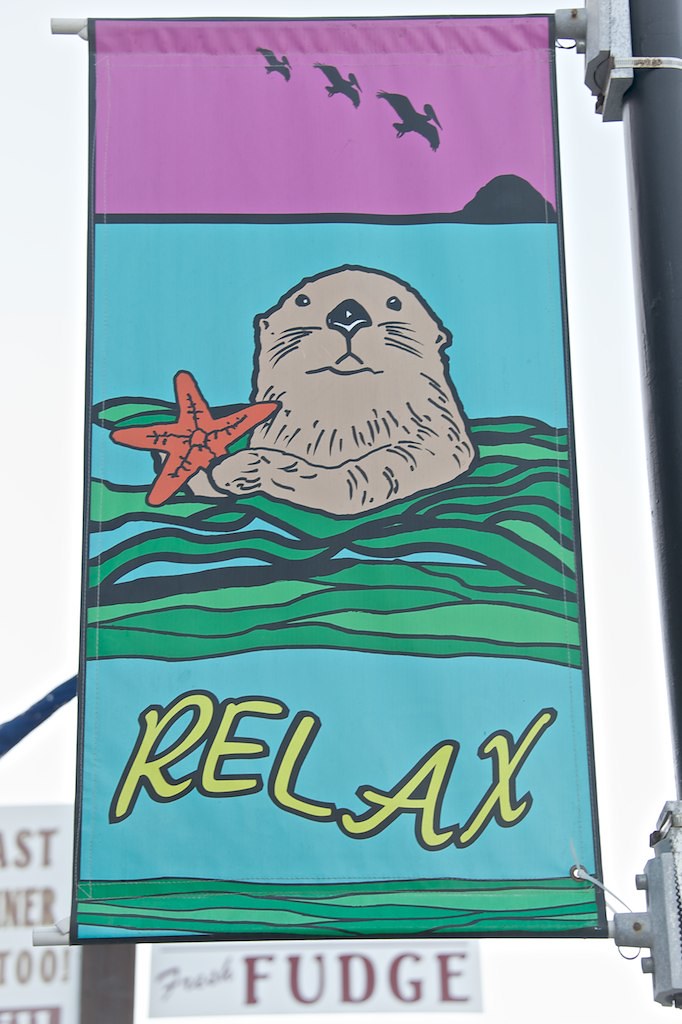The photograph captures a colorful banner prominently displayed on a black metal pole in what appears to be a public place, possibly a street or city square. The banner is affixed to the pole with zip ties, including one hanging at the bottom. The focal point of the banner is a cartoon-like depiction of a brown otter entwined in seaweed, clutching an orange starfish in its paws. Above the otter, the banner transitions into a pink background featuring the silhouettes of three birds, likely seagulls or pelicans, flying against a backdrop that resembles a hill or mountain in black. The sky in the background is white. Below the otter, the word "RELAX" is prominently displayed in wavy green text with a black outline. The lower part of the banner is green, representing kelp. In the blurred background, another placard can be glimpsed, partially legible with the word "fudge," indicating a nearby vendor or shop.